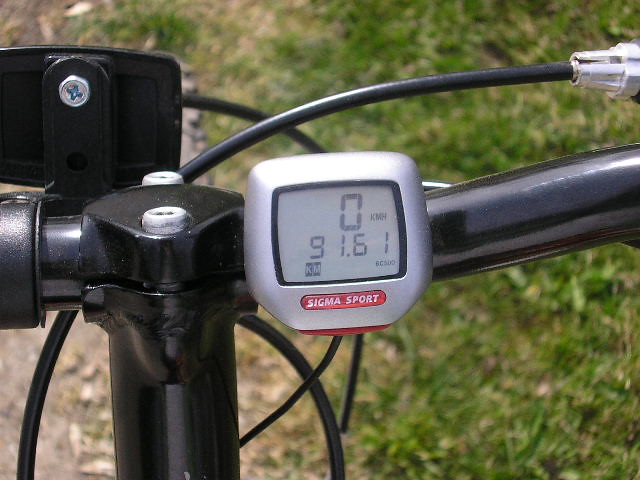This horizontally-aligned, close-up photograph captures the handlebar section of a sleek black bicycle. The focus is on the handlebars, where various wires are prominently extending. Mounted on the handlebar is a small, square, silver digital screen. The screen's background is gray, displaying a black letter "O" and the measurement "91.61 kilometers." Below this, although some text is ineligible, the words "Sigma Sports" are clearly visible, printed in white against a red background. The backdrop of the image features a mixture of green and brown grass, indicating patches of both live and dead vegetation, along with some visible dirt.